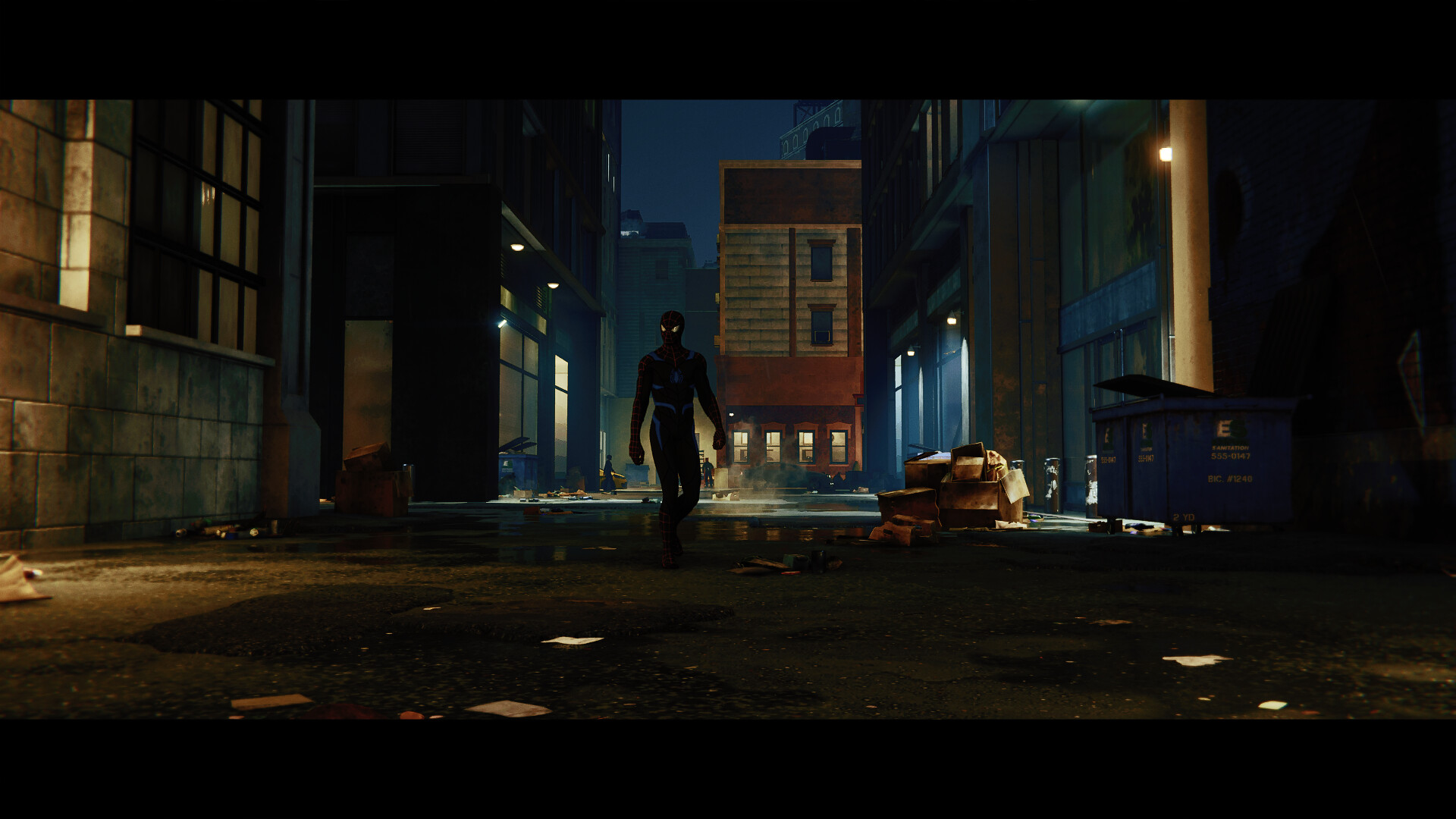This vividly detailed image appears to be a screen capture from a cinematically-styled video game, showcasing a photorealistic, dimly lit cityscape at night. The scene is framed with large black rectangular bars at the top and bottom, resembling the aspect ratio of a wide-screen film on an HDTV. In the center, a character strongly resembling Spider-Man, identifiable by his dark red suit adorned with white lines, a glowing yellow-eyed mask, and a prominent spider logo on the chest, strides purposefully toward the viewer.

To the right of Spider-Man, there is a blue trash can with a black lid set against a backdrop of city storefronts. The storefronts vary in color, with those farthest in the distance being chocolate brown with beige brick linings and those closer being a mix of beige, light gray, and dark gray bricks, alongside a notable blue building closest to him. Scattered around his path on the dark gray pavement are pieces of trash, including cardboard boxes and miscellaneous debris, suggesting an alleyway setting.

The overall atmosphere of the image is dark, with a navy blue night sky overhead and countless dark gray buildings rising in the background. Some light emanates subtly from the windows of the buildings on either side, adding to the moody, nocturnal ambiance of the cityscape. Despite the unclear indications of the specific city, the combination of the urban setting, architectural elements, and the iconic superhero at the center unmistakably conveys a scene of Spider-Man navigating through a shadowed city.